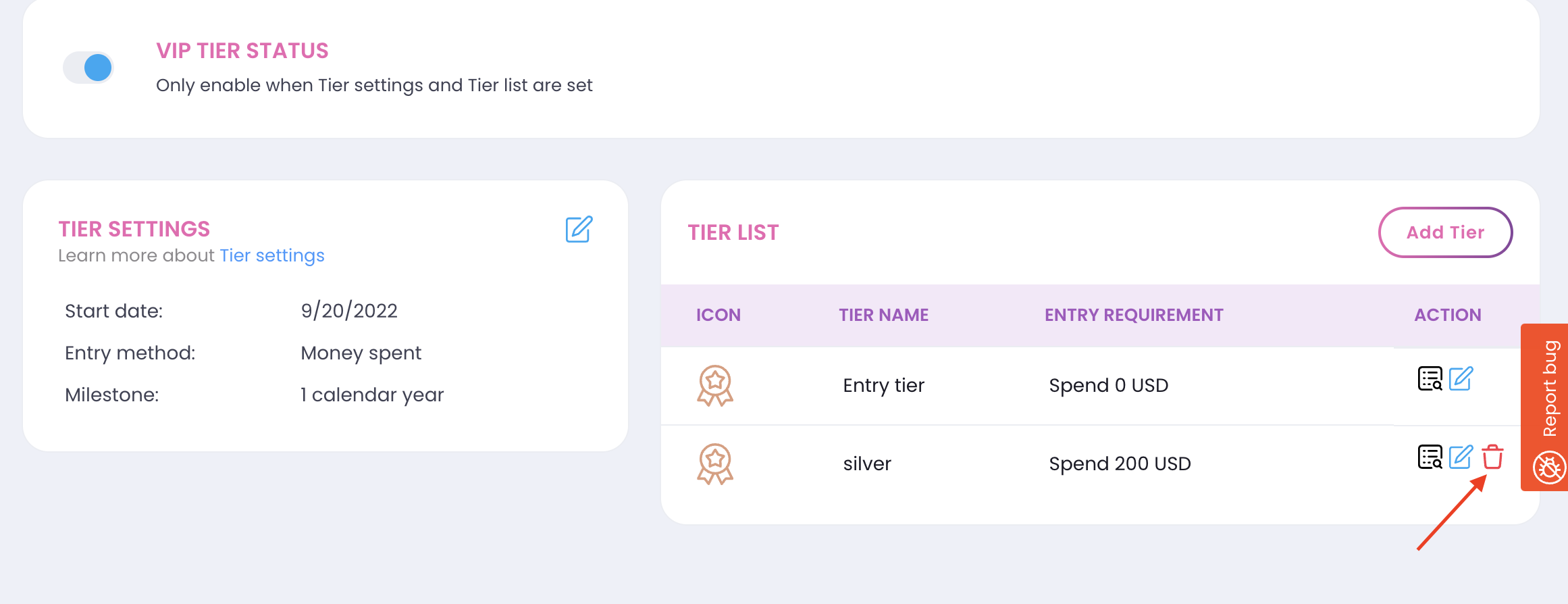In this image, we see a detailed view of a web page interface designed for managing a VIP Tier Status system. At the top of the page, highlighted in pink against a white background, is the heading "VIP Tier Status." Directly below this heading is a toggle switch, which appears to be in the "on" position. The associated instruction, written in black text, reads: "Only enable when tier settings and tier lists are set."

Following this, within a white box, there is an option labeled "Tier Settings," which is designed to be clicked for further information or customization regarding the tier settings. Below this clickable option, several details about the VIP tier program are outlined:

- The start date of the program is listed as "9-20-2022."
- The entry method for the program is defined as "money spent."
- The milestone for maintaining or achieving a tier is set to "one calendar year."

To the right of these details, in pink text on a white background, is another heading labeled "Tier List." Accompanying this is a button for adding a new tier. Under this section, several columns are laid out: "Icon," "Tier Name," "Entry Requirement," and "Action."

The current tiers displayed are:
1. **Entry Tier**
   - Icon: A prize medal
   - Entry Requirement: Spend $0 US dollars

2. **Silver Tier**
   - Icon: A prize medal
   - Tier Name: Silver
   - Entry Requirement: Spend $200 US dollars

Each tier is depicted with a corresponding icon that resembles a prize medal, indicating the tier's prestige.